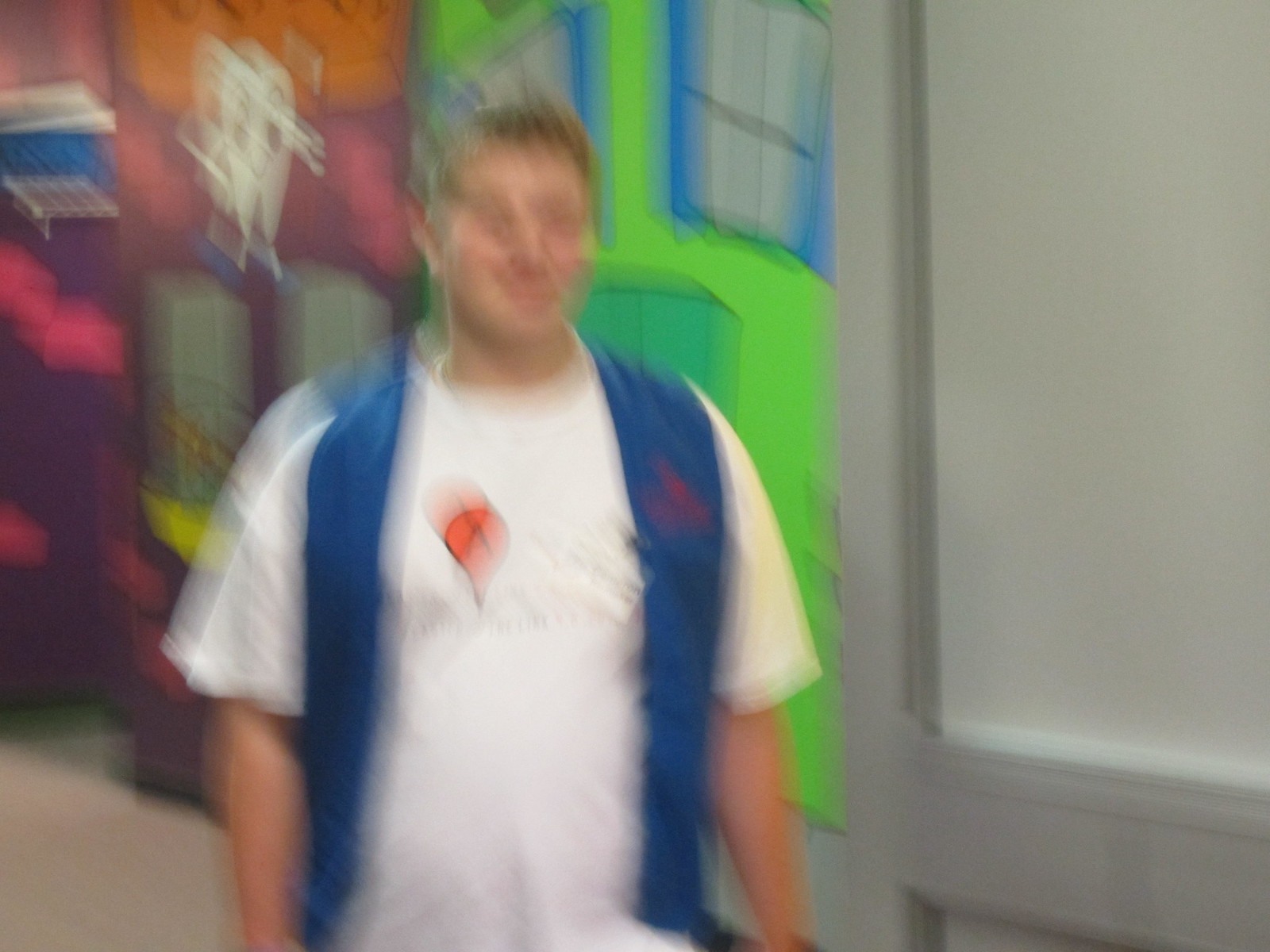A very blurry photograph features a light-skinned man with short, dark blonde hair standing in the center. He wears a white t-shirt adorned with a red Google pin logo featuring the letter "A" and a medium blue vest with a red logo on the front pocket. His arms hang by his sides, and he appears to be smiling slightly. The vibrant backdrop includes a colorful mural depicting a lime green house with blue window panels and a maroon house with yellow window panels. There is a large cartoonized tooth with big eyes and a toothbrush. On the right side of the image is a gray paneled wall.